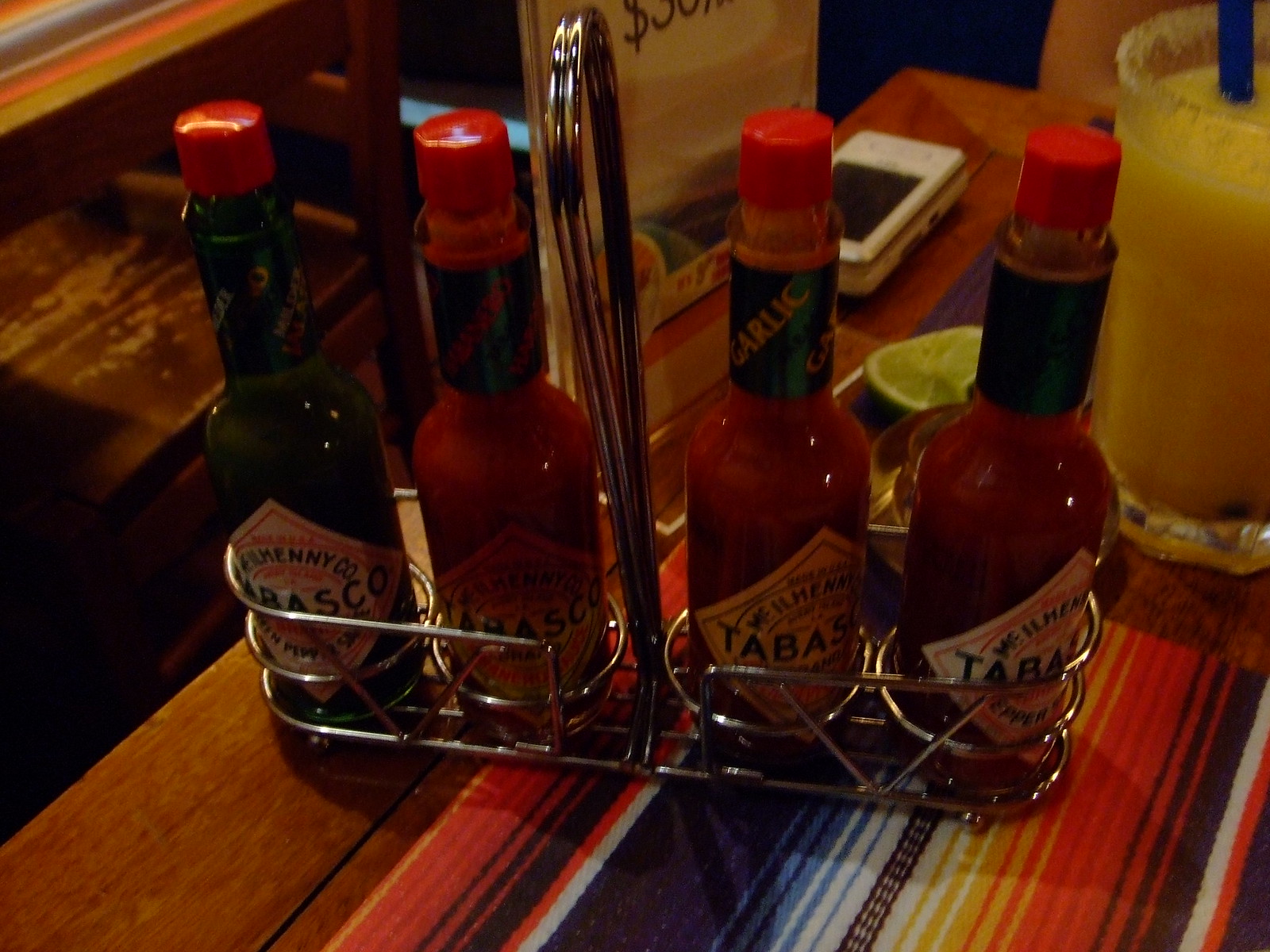In a cozy Mexican restaurant, this close-up captures a rectangular scene of a brown wooden table adorned with a bright, striped tablecloth. Dominating the image is a chrome metal caddy holding four Tabasco bottles. From left to right, the caddy contains a green Tabasco bottle, a blurry red Tabasco bottle of unknown flavor, a red Tabasco bottle with a garlic label, and another red Tabasco bottle of the regular variety. Each bottle is capped with a red top. Just behind the caddy, a refreshing, yellow-orange margarita with salt around the rim and a blue straw peeks into view. An adjacent lime slice lies on the table near a bulky, white object that looks like an early 2000s cell phone or another nostalgic tech device, possibly a pocket tape recorder. Adding to the ambiance, a plastic standee displaying a partially visible ad with a dollar sign stands in the background, encapsulating the vintage, eclectic charm of the scene.